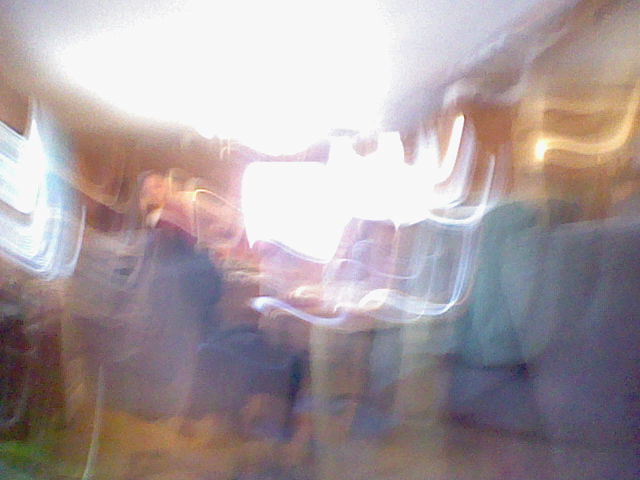This exceedingly blurry image features extreme motion blur, suggesting that the camera was either dropped or jerked sharply. The scene appears to be set in a kitchen, identified by the presence of brown cabinets and a window allowing an influx of natural light. The blur swirls this light around the image, further disguising the details. Amidst the blur, a figure can partially be seen, either sitting on a chair or standing in the kitchen. Their facial features, however, are stretched and indistinct due to the motion blur.